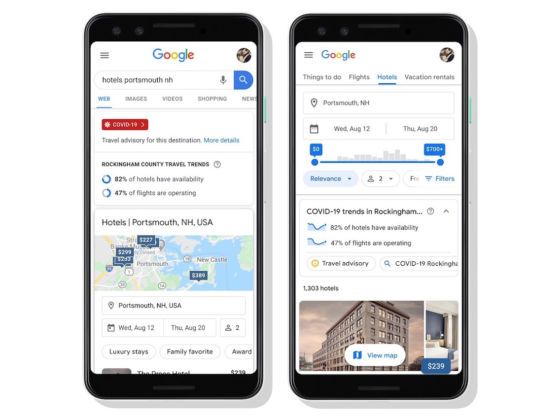In this image, we observe two smartphones placed side by side, both displaying search results from Google. The phone on the left shows a search query for "Hotels Portsmouth NH." The search results highlight a COVID-19 travel advisory specific to the destination, along with travel trends for Buckingham County. Key statistics include 82% hotel availability and 47% of flights operating. Additionally, the search results feature a map of Portsmouth, NH with various hotels marked by blue rectangles displaying their respective prices.

The phone on the right is set to the "Hotels" tab with the location input as Portsmouth, NH. The specified travel dates range from Wednesday, August 12th to Thursday, August 20th, and the price range filter is set from $0 to $700+. This search results page also includes COVID-19 trends, indicating there are 1,303 hotels available. Beneath this, there is an image of the exterior of a hotel and a photo of one of the interior rooms, giving a visual representation of potential accommodations.